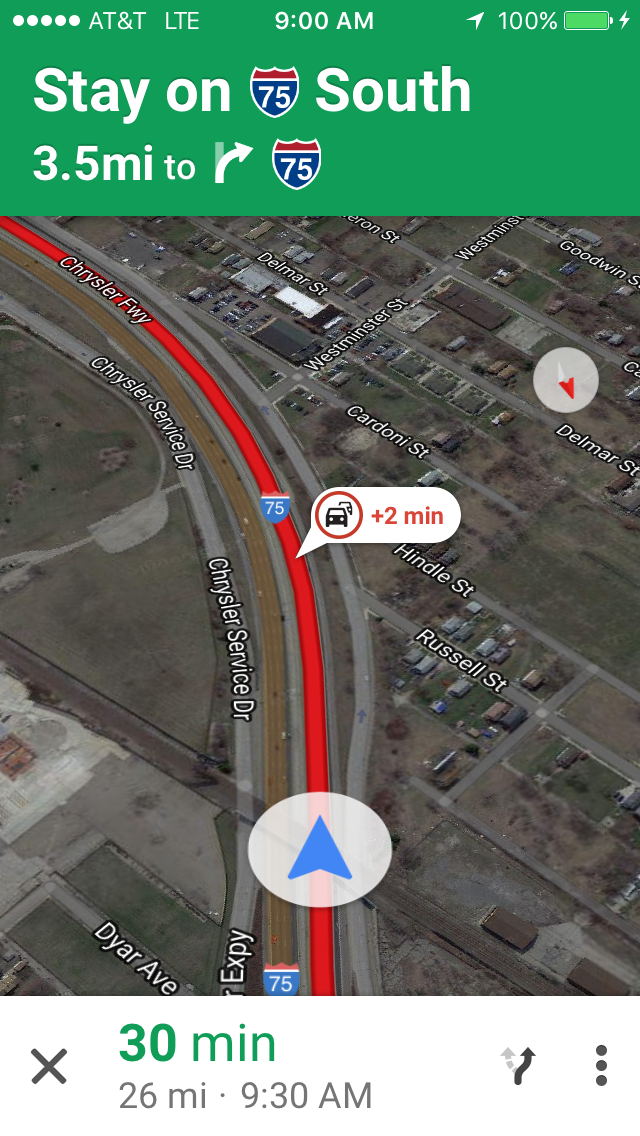The image is a detailed screenshot from a mobile phone displaying GPS navigation on a city map. At the top of the screen, the phone indicates it is 9 AM with AT&T LTE service and a full battery. The map instructs the user to stay on I-75 South for 3.5 miles and then to make a right on I-75. The route includes various points of interest such as Chrysler Service Drive, Chrysler Parkway, Russell Street, Hindle Street, and Dyer Avenue. The map also highlights a traffic delay due to an accident ahead, adding 2 minutes to the journey, and shows traffic conditions using colors like red, blue, white, gray, and bright green. The expected time of arrival (ETA) is 9:30 AM, with a total distance of 26 miles remaining. Satellite imagery shows the highway passing through an urban area with homes and streets prominently displayed. The overlay includes details such as street names, highway numbers, arrows for directions, and traffic alerts, creating a comprehensive navigational display reminiscent of a day-time scenario.